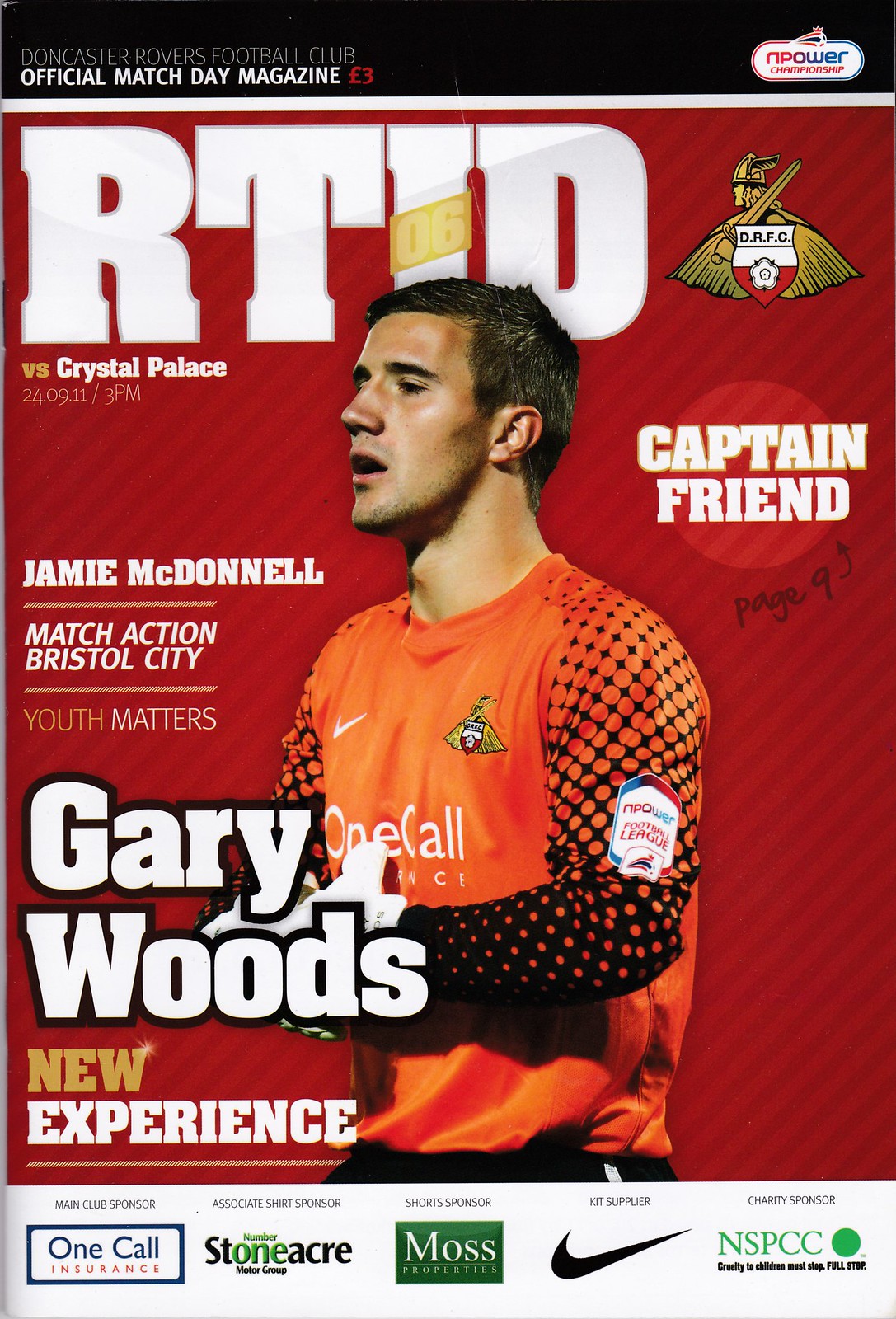The advertisement image features a soccer player prominently superimposed over a striking red background with darker red stripes. The player, a white male with short brown hair and brown eyebrows, faces to the left with an open mouth, possibly mid-sigh or in intense concentration. He is dressed in an orange uniform that fades into a beehive pattern of polka dots on the black sleeves. This dynamic scene is framed by various text elements: at the top, a black banner reads, "Nontaster Rovers Football Club Official Match Day Magazine." Just below, in the red area right above his head, large white letters spell out "RTID." 

Additional text details the content and sponsors: to his left, bold white and black-outlined text announces, "Gary Wood's new experience." Other informative captions include, "Jamie McDonald, Match Action," "Bristol City Youth Matters," and "RTID versus Crystal Palace, 2-49-09-11-3pm." In the top right corner, a gold symbol of a man with a sword, cape, and helmet accompanies the circular white text stating, "Captain Friend." At the bottom stripe, which is white, various sponsors are listed, including, "One Call Insurance," "Number Stone Maker," "Moss Properties," "Nike," and the charity, "NSPCC," emphasizing their cause, "Cruelty to Children Must Stop, Full Stop." The overall vibrant and detailed design captures dynamic action while effectively promoting the event and its sponsors.